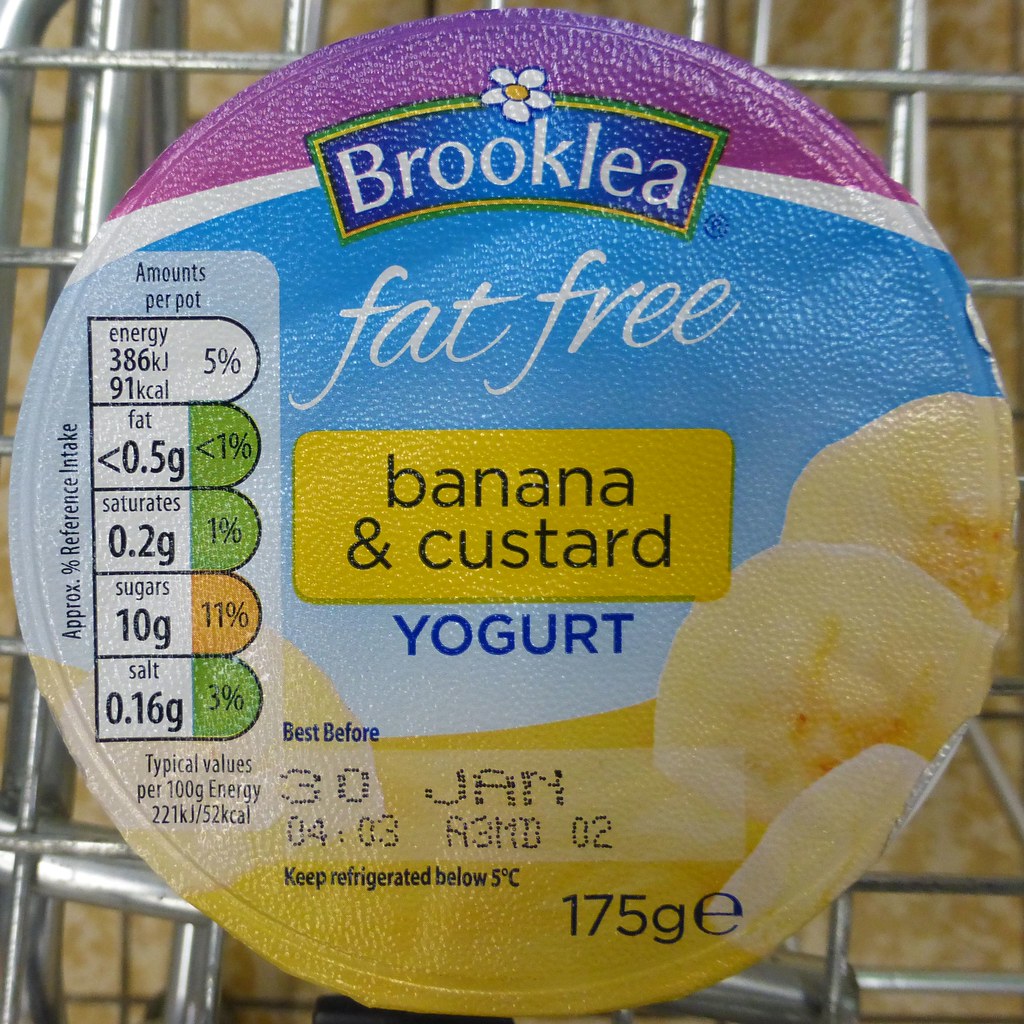This photograph depicts a Brooklia fat-free banana and custard yogurt container. The container is primarily purple with some blue accents and features a yellow background on the lid, which displays lifelike images of bananas and custard. The label reads "Brooklia Fat-Free Banana and Custard Yogurt" in a combination of white and black text. It specifies a "Best before 30th January 0403 A3 MD02" date and advises to "Keep refrigerated below 5°C." The lid is slightly peeling on the right side, but the yogurt appears unopened and intact. The package contains 175 grams of yogurt, with nutritional information on the left, detailing amounts of fat, saturates, sugars, and salts, with salt listed at 3%. The yogurt container is placed on a metal cooling rack that sits atop a brown countertop. The scene suggests it's part of a grocery shopping experience, given the presence of a shopping cart in the background.